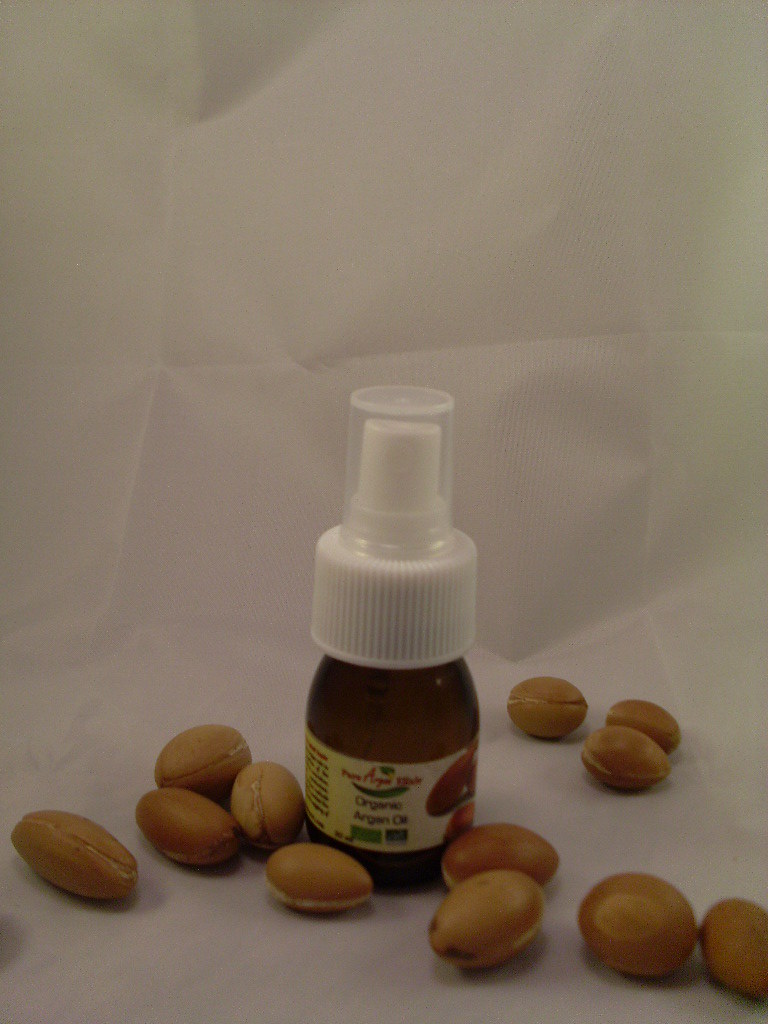This photograph features a small, one-ounce, brown bottle of organic argan oil with a spray top, covered by a clear plastic lid. The bottle is set against a white background that appears to be a piece of folded paper. The label is white with green, yellow, brown, and red lettering, displaying the text "organic argan oil" along with some ingredient details on the side. Surrounding the bottle are approximately twelve small, brownish, oval-shaped objects, likely argan seeds or nuts. The image is dark and has a muted color palette, with no visible date, name, or person included.